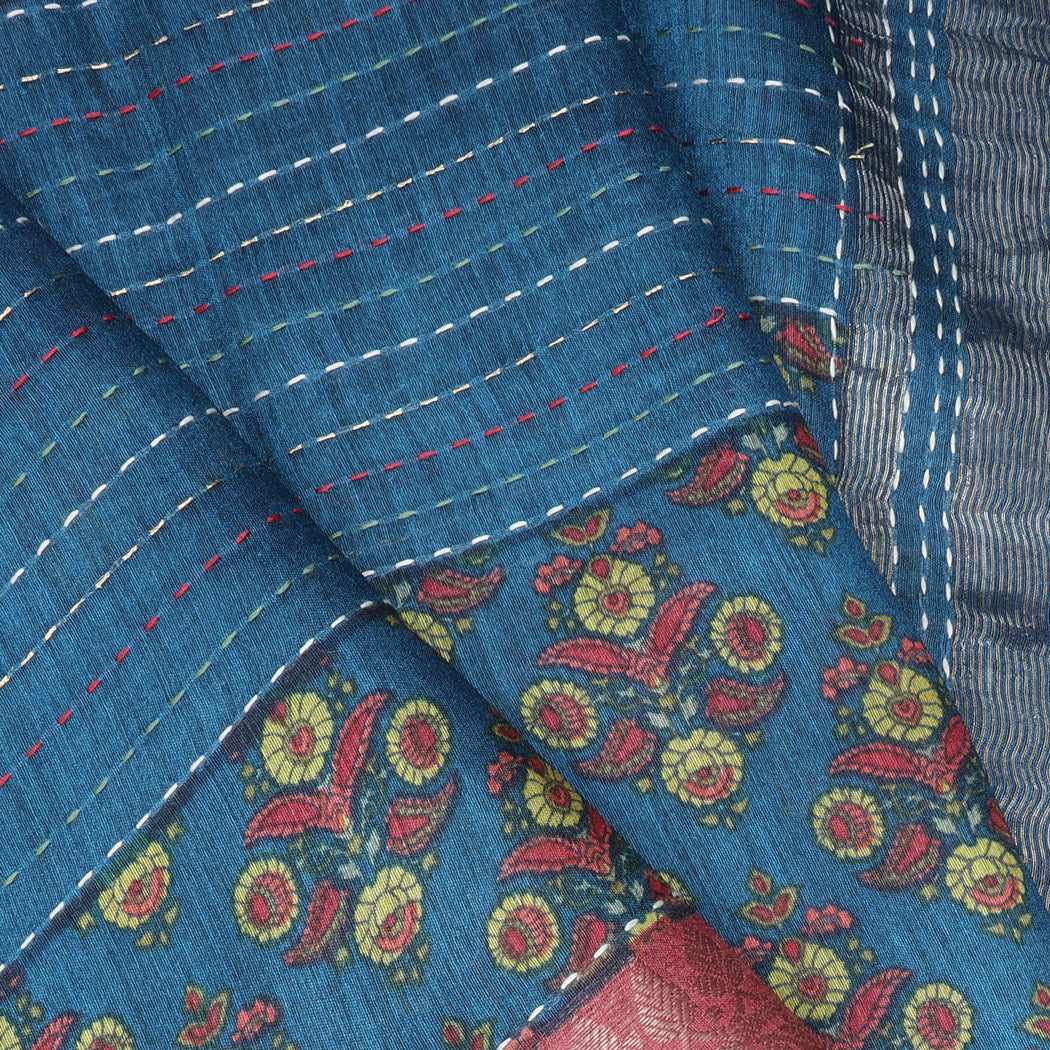This highly detailed close-up image features a meticulously crafted quilt composed of various fabrics in shades of blue, red, yellow, and white, which is folded over itself to fill the entire frame. The upper left-hand corner prominently displays rows of intricate hand-stitching, alternating in colors: white, yellowish-green, and red. The stitches, spaced about half an inch apart, create a captivating pattern that enhances the quilt's texture.

Further down the quilt, a section adorned with vivid floral patterns emerges. The flowers showcase yellow petals with red centers, framed by paisley designs that include red elements centered within each set of four flowers. This floral panel transitions into another segment, where a red fabric with a leaf-textured pattern stands out, adding depth to the composition.

Contrasting reports also mention that the quilt resembles blue jean material adorned with embroidered white, cream, burgundy, and green lines, rotating down the fabric. Additionally, the embroidery includes burgundy leafing and yellow flowers with burgundy centers, suggesting a consistent theme of floral and leaf motifs.

At the very bottom, there is a solid burgundy matte fabric panel, contributing to the rich tapestry of textures and colors. This section reinforces the quilt's stunning craftsmanship, making it a profound piece that elegantly combines various elements and intricate details.